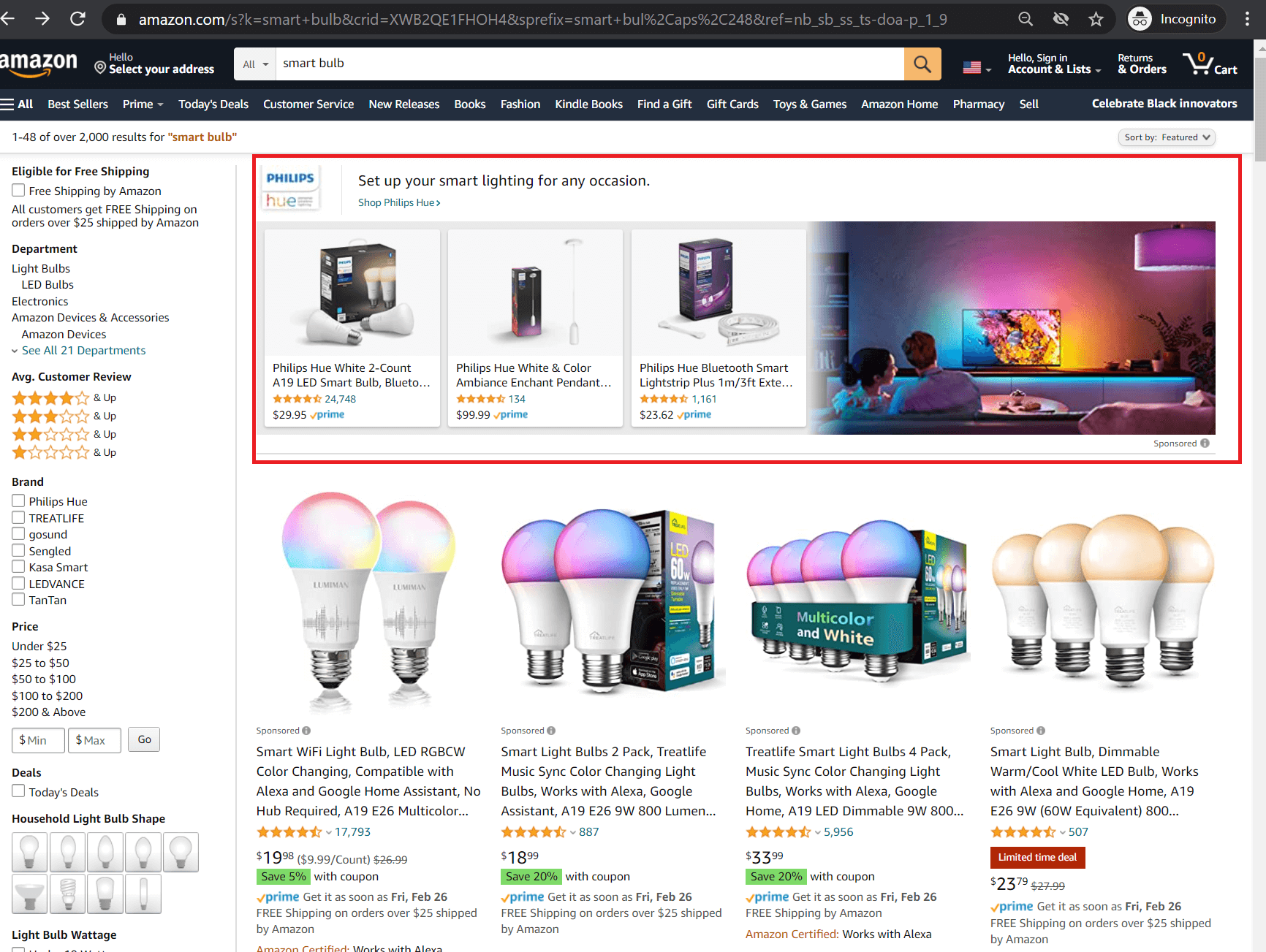This image depicts an Amazon shopping page for an account. At the top of the interface, there is a charcoal gray navigation bar featuring white text and directional arrows pointing left and right. To the left of this navigation bar, there is a padlock icon indicating a secure connection, adjacent to a search bar containing the Amazon web address. To the right of the web address, a white magnifying glass icon is present, followed by icons representing bookmarked favorites and incognito mode. At the far right of this bar, there are three vertical white dots, representing a menu.

Beneath this, the Amazon logo appears on the left, followed by an option to select your address. This is accompanied by a broad, white search bar. At the right end of this search bar, there is a yellow button featuring a black magnifying glass for initiating searches. Continuing to the right, there is an American flag icon with a drop-down menu for selecting regional settings, followed by links for "Accounts & Lists," "Returns & Orders," and a cart icon indicating items in the cart.

Below this, the product search results for "Smart Bulb" are displayed. The results headline reads "Philips, set up your smart lighting for any occasion," and showcase multiple bulb options, including Bluetooth-connected lights.

At the bottom of the page, four distinct product results are visible: the first item is a set of Smart Wi-Fi Light Bulbs (LED), the second item is a set of smart light bulbs with color-changing capabilities, the third is a four-pack of bulbs, and the fourth offering features dimmable bulbs.